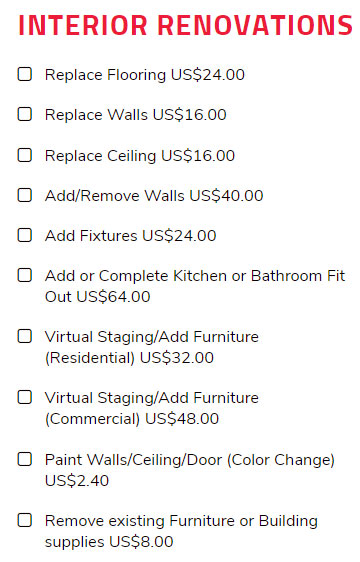Here is the cleaned-up and detailed caption:

---

A detailed list titled "Interior Renovations" at the top in red lettering, indicating various renovation tasks, each with a corresponding checkbox and cost. The list is divided into individual lines of black text and includes the following items with specified costs:

1. Replace flooring - US $24
2. Replace walls - US $16
3. Replace ceiling - US $16
4. Add/remove walls - US $40
5. Add fixtures - US $24
6. Complete kitchen or bathroom fit-out - US $64
7. Virtual staging/add furniture (Residential) - US $32
8. Virtual staging/add furniture (Commercial) - US $48
9. Paint walls/ceiling/door (Color change) - US $2.40
10. Remove existing furniture or building supplies - US $8

Given the unrealistically low prices for these extensive renovation tasks, it appears this list might be from a video game or a virtual simulation, rather than a real-life context. There are no additional details, hyperlinks, or website addresses provided.

---